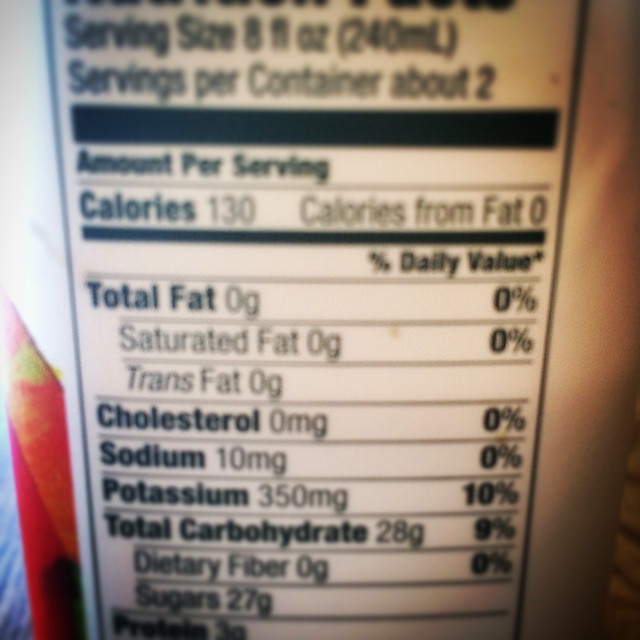The image is a blurry, close-up photograph of a nutrition label on a can. The label presents detailed dietary information, though parts of it are out of focus. At the top, the serving size is listed as 8 fluid ounces (240 milliliters), with approximately 2 servings per container. It states the amount per serving, showing 130 calories, with 0 calories from fat. The detailed nutritional facts include 0 grams of total fat, saturated fat, and trans fat, 0 milligrams of cholesterol, 10 milligrams of sodium, 350 milligrams of potassium, and 28 grams of total carbohydrates. These carbohydrates consist of dietary fibers and sugars, though the precise amounts may be partially obscured by the blurriness of the image.